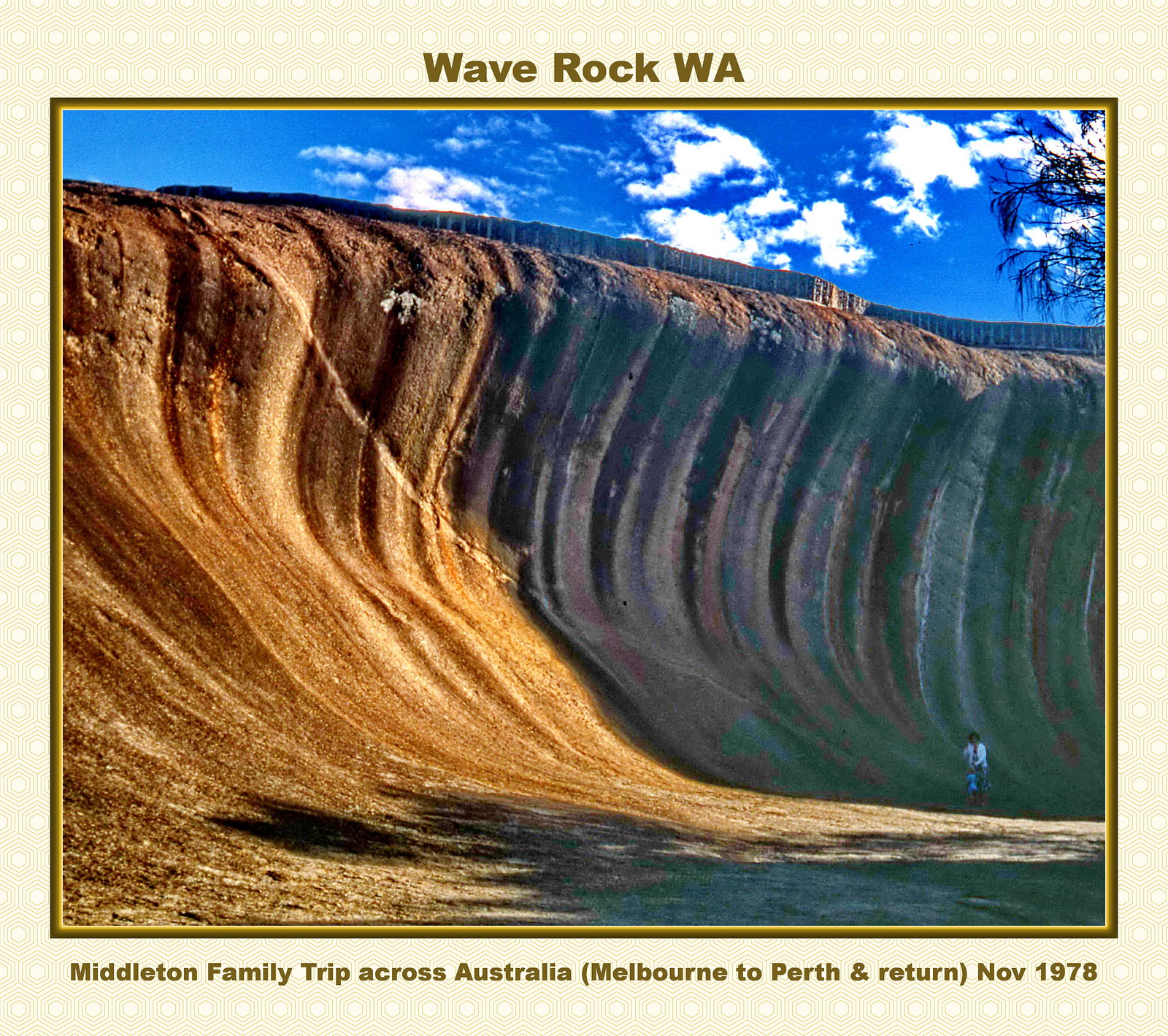This vibrant photograph, captioned "Wave Rock WA" in gold font on a cream background at the top, depicts the iconic Wave Rock in Western Australia. The rock formation, resembling a giant wave frozen in time, showcases a stunning mix of light and dark brown hues, along with beige and white striped patterns running vertically. The rock curves inward and outward, creating a sense of movement akin to a cresting wave. A tiny figure, wearing what appears to be a white shirt, stands at the bottom right, accentuating the immense scale of the formation. Above, the sky is partly cloudy, with vibrant blue tones and scattered white clouds, and a tree limb juts into view from the top right corner. At the bottom of the image, the text reads, "Middleton family trip across Australia, Melbourne to Perth and return of 1978" in the same gold font. The entire photograph is bordered by a gold frame, adding a touch of elegance to this striking visual memoir from the Middleton family's 1978 journey.